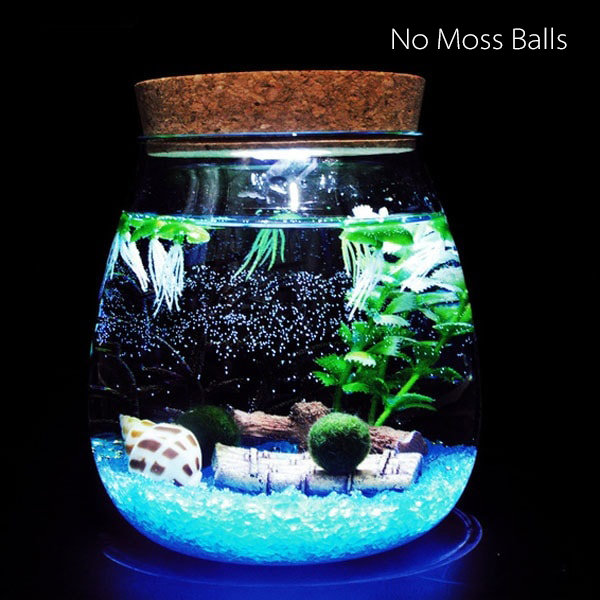This image depicts a meticulously crafted water diorama set against a stark black background, accentuated with studio lighting for a modern, polished appearance. At the center of this square photo lies a rounded, square-shaped glass jar sealed with a cork lid. The jar, filled approximately seven-eighths with water, houses a miniature underwater scene, evocative of a treasure-laden seascape.

Inside the jar, clusters of green plants imitate the appearance of jellyfish, their tendrils reminiscent of Medusa's locks. These jellyfish-like plants float near the top, enhancing the underwater illusion. Alongside them, nondescript green plants provide additional texture in the background.

At the base of the jar, blue crystals mimic the ocean floor, supporting a small, white shell adorned with brown rectangles, reminiscent of a sea snail. Resting on a fake treasure chest is a vivid green moss ball, contrasting with the surrounding elements. A piece of driftwood adds to the natural aesthetic.

Curiously, white text in thin letters at the upper right-hand corner reads, "No Moss Balls," which juxtaposes the presence of the moss ball inside the jar. This diorama, likely a collector's item or a handmade creation similar to those found on Etsy, is a captivating blend of aquatic charm and creative artistry.